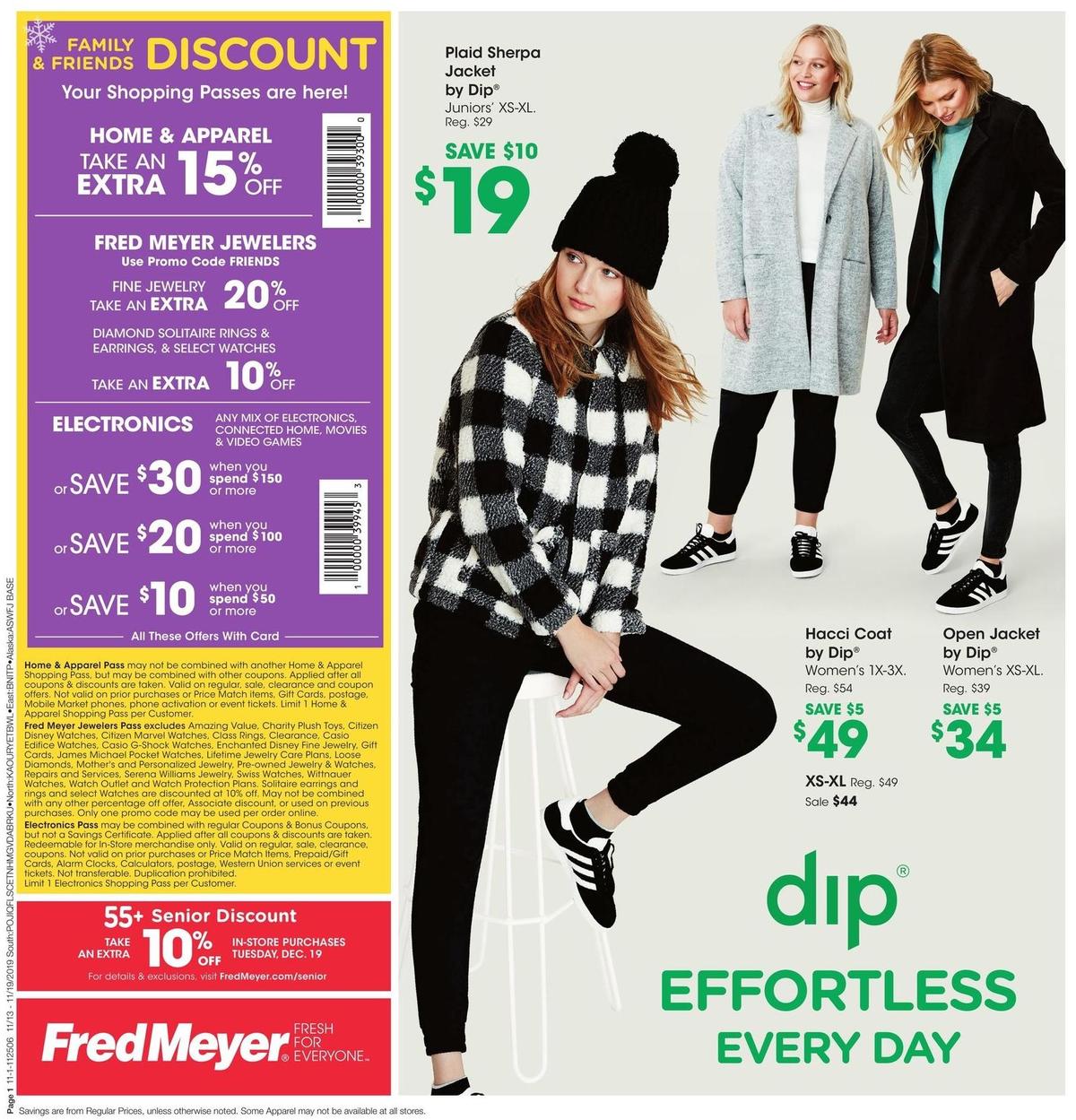Certainly! Here is a cleaned-up and detailed caption for the image you described:

---

**Fred Meyer Web Page Advertisement**

This web page showcases multiple shopping discounts and offers from Fred Meyer. On the left side, there is a detailed navigation column listing various promotions and discount categories, including:

- Fred's Discount: Family and Friends Discount
- Shopping Passes: Extra savings on home and apparel with an additional 15% off Fred Meyer Jewelers using promo code 'FRIENDS.'
- Fine Jewelry: Extra 20% off Diamond Solitary Rings, Earrings, and select Watches.
- Electronics: Various offers such as an extra 10% off an assortment of electronics, including connected home devices, movies, and video games. Additionally, save $30 when you spend $150 or more, $20 when you spend $100 or more, or $10 when you spend $50 or more, all with the use of a Fred Meyer card.
- Senior Discount: Customers aged 55 and above can take an extra 10% off in-store purchases on Tuesday, December 19th.

Barcodes for scanning at checkout are provided at the bottom of the page.

On the right side of the page, there is an advertisement featuring three models showcasing winter apparel. All three models are wearing the same stretchy black pants paired with identical black shoes that have white stripes on the side. Each model sports a different coat:
- The first model wears a plaid Sherpa jacket on sale for $19.
- The second model is in a herringbone coat priced at $49.
- The third model wears an open-front jacket priced at $34.
- One model also sports a black beanie with a large pom-pom on top.

The advertisement is captioned with "Dip: Effortless Every Day" at the bottom, emphasizing the brand’s commitment to casual and easy-to-wear fashion.

Fred Meyer’s tagline, "Fresh for Everyone," is also prominently displayed.

---

This detailed caption offers a comprehensive overview of the content and promotions featured in the image.